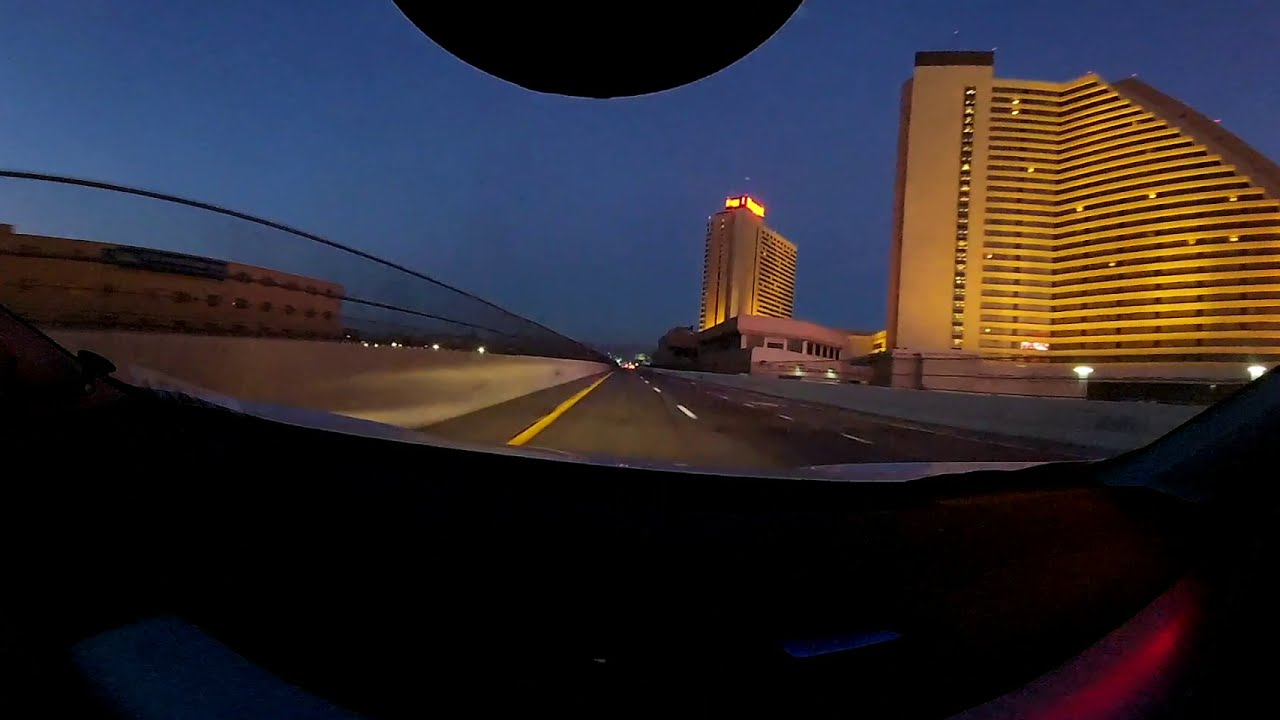Captured through the windshield of a sporty car driving at night, this image showcases a nearly desolate stretch of a three-lane freeway. The car is positioned in the leftmost lane, adjacent to a barrier. Towering on the left side beyond the barrier is a three-story building that exudes a somewhat eerie, prison-like appearance. Meanwhile, to the right side of the road, two prominent, modern buildings rise against the twilight sky. One of these buildings features a distinctive, graduated pyramid structure that narrows at a 45-degree angle as it ascends, possibly a high-rise hotel or luxury apartments. The dusk is setting in, painting the sky in hues of blue turning gray and purple, while lights begin to illuminate the scene. The sphere protruding from the upper middle of the photo is likely a component of the car. Traffic is sparse, contributing to the serene, almost isolated ambiance of what appears to be a Sunday evening. Despite the diminishing daylight, the area is strikingly calm and largely unpopulated.